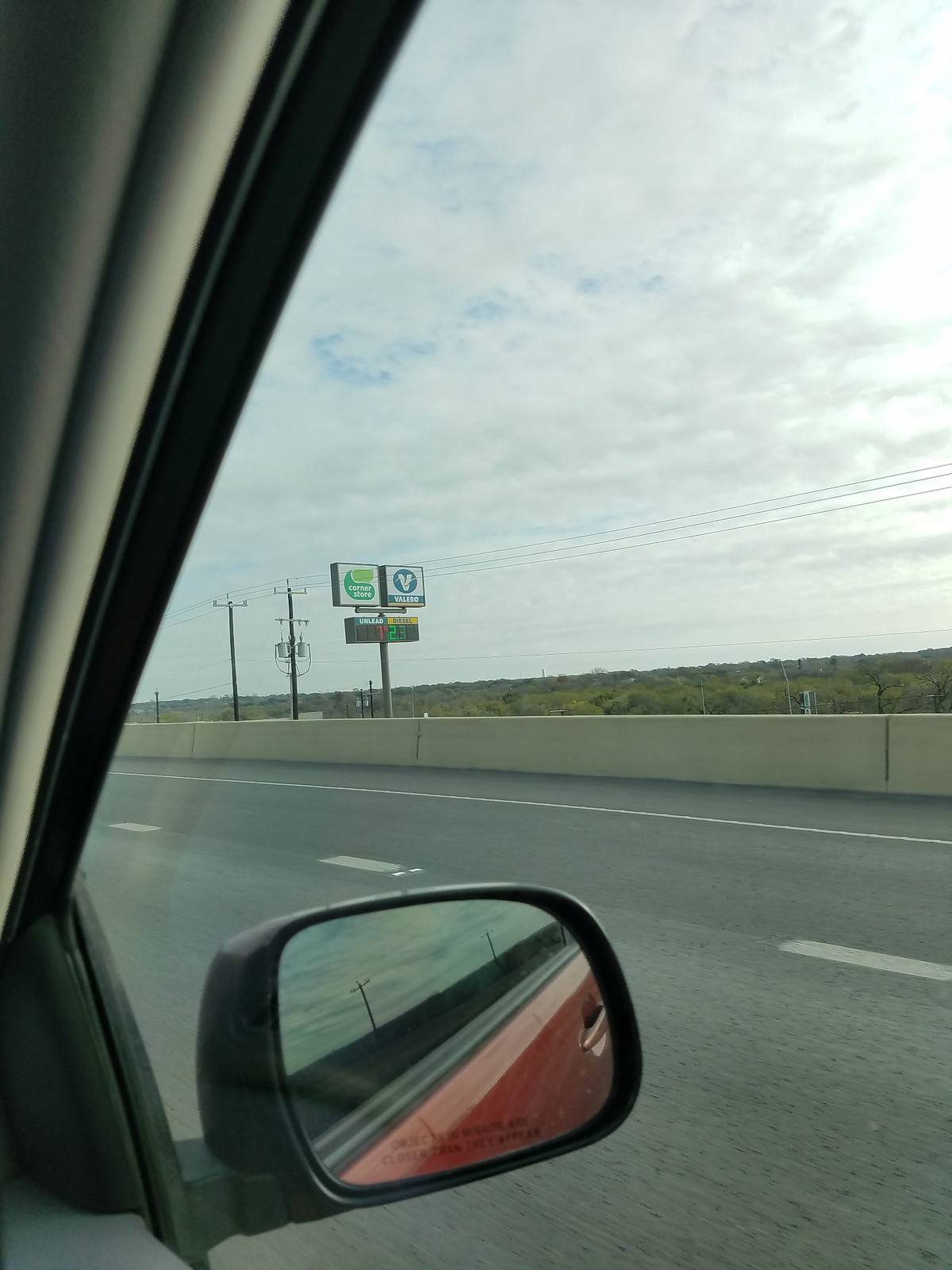A dynamic photograph captured from within a moving vehicle, gazing out of the passenger side window. The image prominently features the paved road on which the vehicle travels, flanked by a robust concrete barrier on the roadside. Beyond this barrier lies a stretch of indistinct vegetation, blurred by distance. Overhead, the sky is a mix of overcast clouds and sparse patches of blue, adding a touch of color to the otherwise grayish scene. In the middle distance, several billboards mounted on tall poles come into view. Among these billboards, three distinct signs are visible; one is positioned at the bottom, while two others are installed higher up.